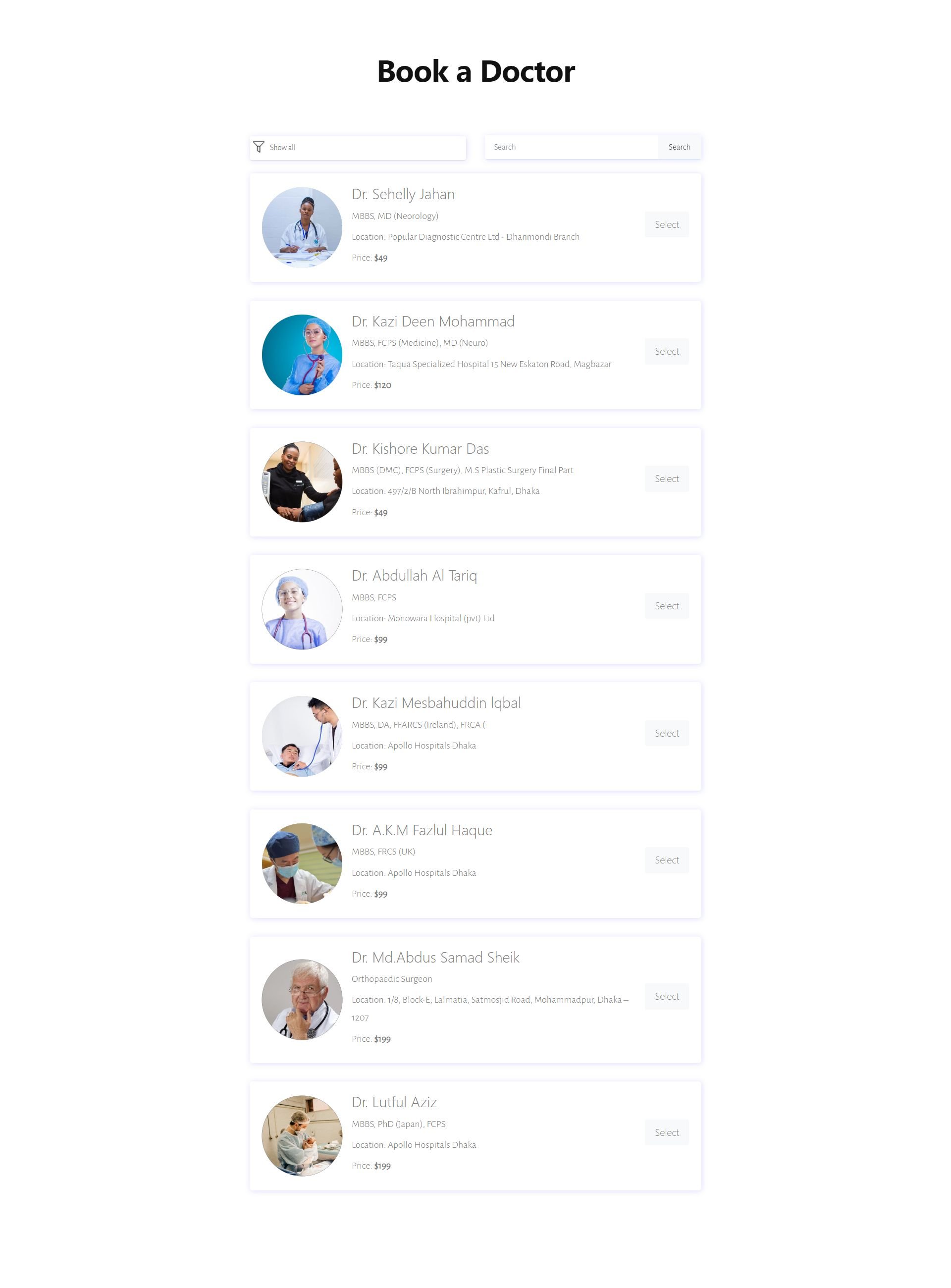The image is a screenshot of a website, predominantly showcasing a booking interface for doctor appointments. The site features a clean, white background, likely indicating a mobile-friendly design due to its vertical layout. 

At the very top of the page, bold black text prominently reads "Book a Doctor". Immediately beneath this heading are two light gray search fields, which contain some indiscernible text - either due to the low-resolution quality of the screenshot or because the text is faint and difficult to read.

Following these search fields, there are listed profiles of doctors, each encapsulated within a white rectangle:

1. **Dr. Shelly Jahan**: This entry is accompanied by a circular photo of an Indian woman clad in professional medical attire, complete with a stethoscope draped around her neck, emphasizing her role as a physician.

2. **Dr. Kazi Dean Mohammed**: Positioned below Dr. Jahan, this listing includes a circular photograph of a Middle Eastern woman dressed in medical scrubs, suggesting her readiness for clinical work.

3. **Dr. Kishore Kumar Das**: The final entry visible in the screenshot features a circular image of a Middle Eastern man dressed casually in a black tracksuit, standing out from the more traditionally attired medical professionals above.

Overall, the image is a functional representation of a user interface designed to facilitate the booking of medical appointments, despite the low-quality visualization of its finer details.